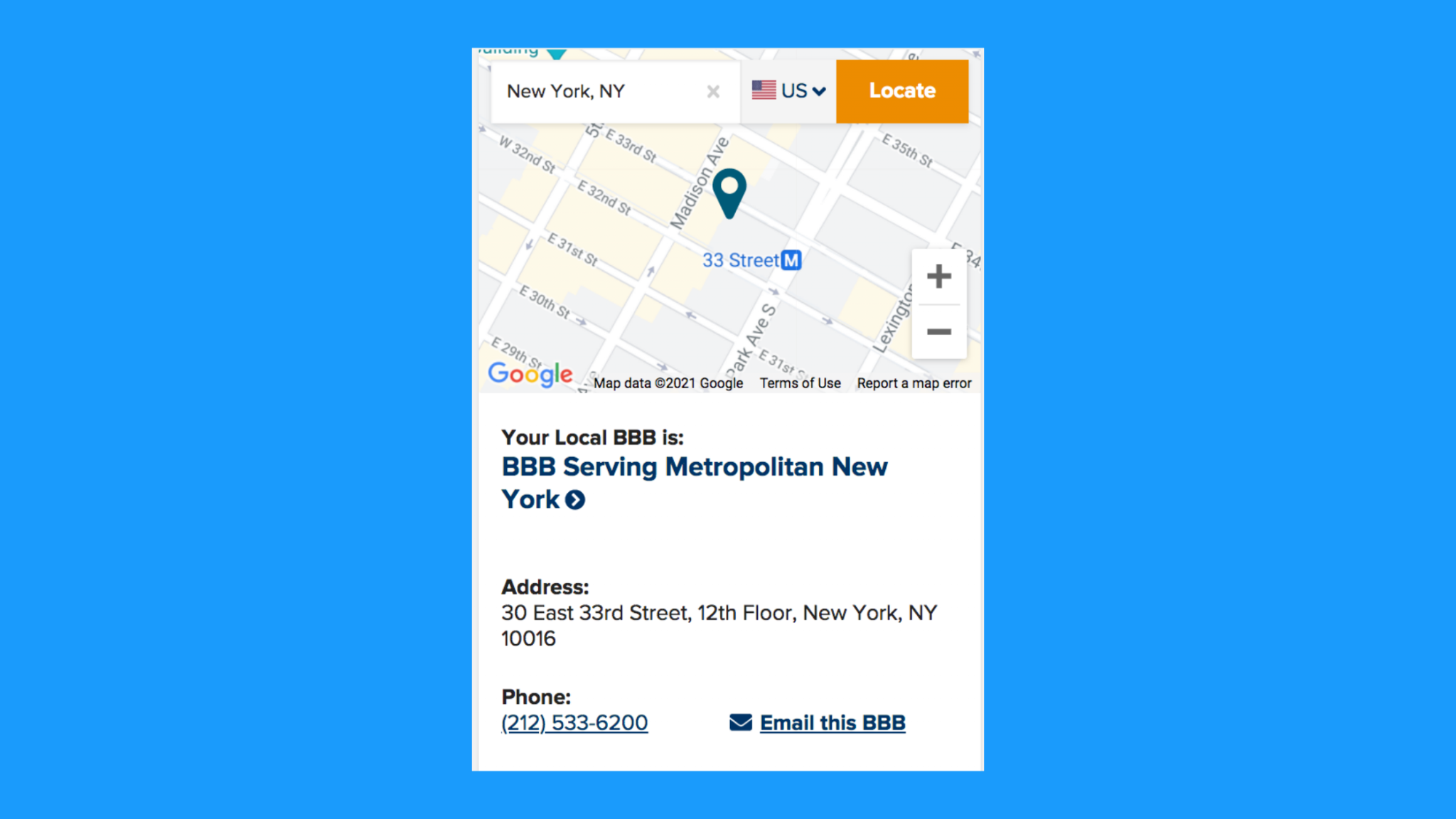This is a detailed description of a Google Maps screenshot showcasing the location of the Better Business Bureau (BBB) serving Metropolitan New York. 

The screenshot features a map overlaid on a sky-blue background occupying roughly 60% of the image. The map displays a section of New York City, with the search box labeled "New York" located in the upper left corner. A light gray "X" icon allows users to clear the search term. To the right, there is a dropdown menu with an American flag and the text "US," followed by an orange button labeled "Locate."

The center of the screenshot reveals a grid layout of the city's streets. The streets include East 35th Street, East 34th Street (unlabeled), East 33rd Street, East 32nd Street, East 31st Street, East 30th Street, and East 29th Street. A green location icon is positioned near East 33rd Street, indicating the BBB's exact location. Additionally, there is a blue box with a white "M" symbol near Park Ave South, resembling a Metro icon. Park Ave South is a major street running diagonally toward the upper right (northeast).

Typical Google Maps features such as zoom in and out buttons are located in the bottom right corner, while the "Google" text appears in the bottom left. The map includes copyright information, terms of use, and a prompt to report a map error.

Below the map, on a white background, the BBB's details are provided. The text reads: "Your local BBB is BBB serving Metropolitan New York," with "York" on a new line. To the right, there is a blue circle containing a bracket symbol. The address provided is "30 East 33rd Street, 12th Floor, New York, New York, 10116." At the very bottom, contact information is listed as follows: 

Phone: (212) 533-6200

An email icon in dark blue indicates an email option, with the text "Email this BBB" underlined and bolded. 

This comprehensive description captures all the elements visible in the screenshot, providing readers with a clear understanding of the image's content.